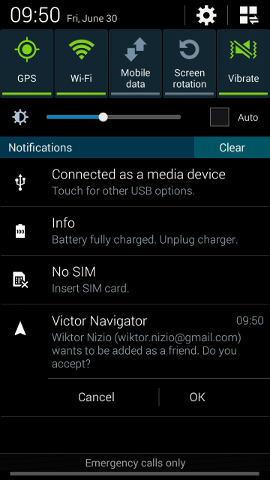The image is a screenshot of a smartphone's pull-down notification bar. At the top left corner, the time is displayed as 9:50 AM. To the right of the time, the date is shown as Friday, June 30th. The first notification below the date indicates that the device is "Connected as a media device" with a prompt to "Touch for other USB options."

Further down, another notification reads "Battery fully charged." Below this, there is a notification stating, "No SIM card," prompting the user to "Insert SIM card."

Additionally, there is a notification from an app or service named Victor Navigator. This notification informs the user that "Victor Enzio wants to be added as a friend." There are two action buttons available: "OK" on the right and "Cancel" on the left.